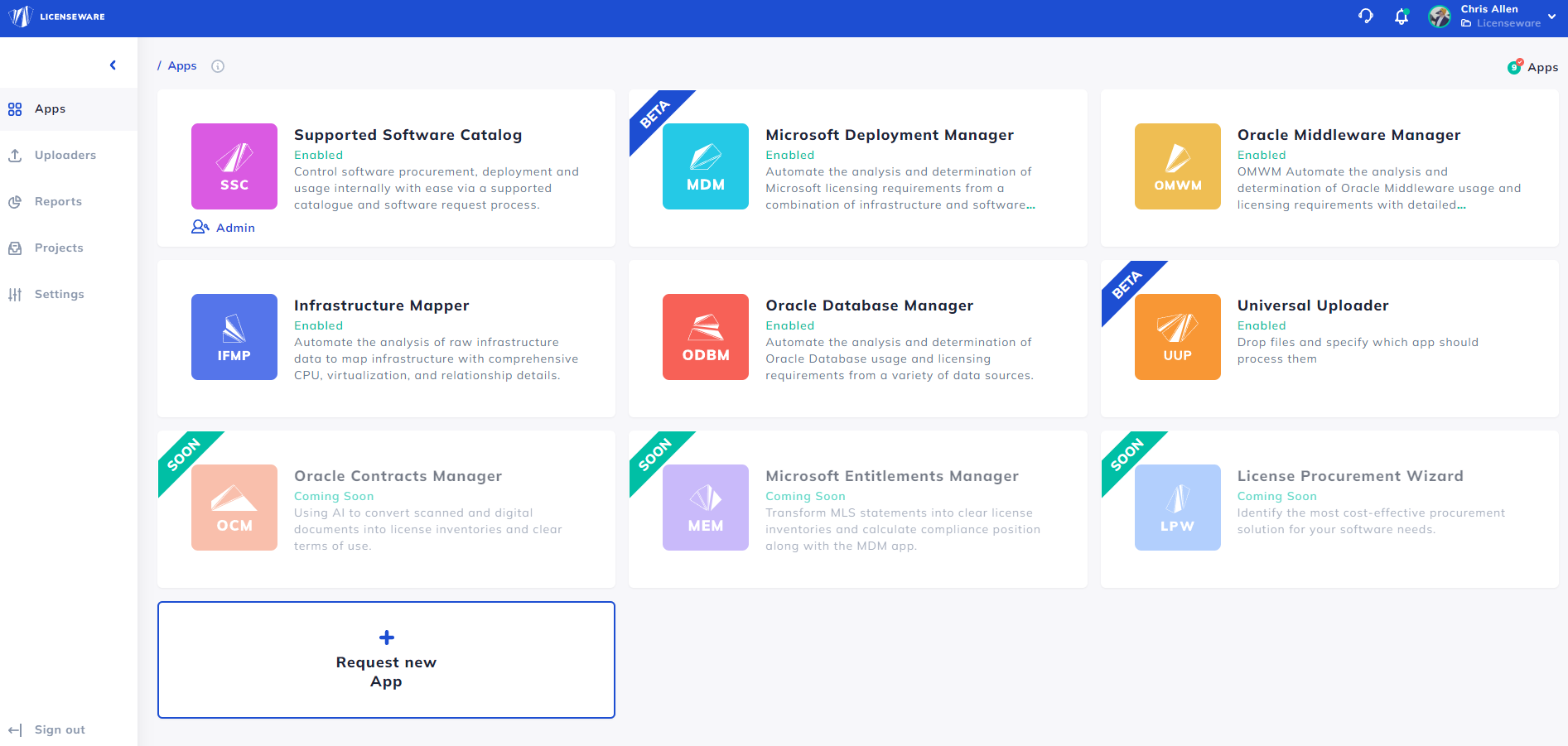This image depicts a web page with a variety of software tools listed. 

The text on the page is quite small, making it difficult to read, even when enlarged in the Chrome browser. 

In the upper left corner, there's a small purple square with the acronym "SSC" inside, which stands for Supported Software Catalog. 

Directly below SSC, there is another square labeled "Infrastructure Mapper" (IFMP). Below that is an "Oracle Contacts Manager" (OCM), which is accompanied by a light orange square. 

In the top center, a light greenish-blue square signifies the "Microsoft Deployment Manager" (MDM). 

The central part of the page features a red square labeled "ODBM," representing the Oracle Database Manager. 

Below ODBM, the "Microsoft Element Manager" (MEM) is marked by a purplish square. 

Further down, there's a yellow square labeled "Oracle Midware Manager". 

An orange square beside it identifies the "Universal Uploader". 

Finally, in the bottom right corner, a blue square indicates the "License Procurement Wizard".